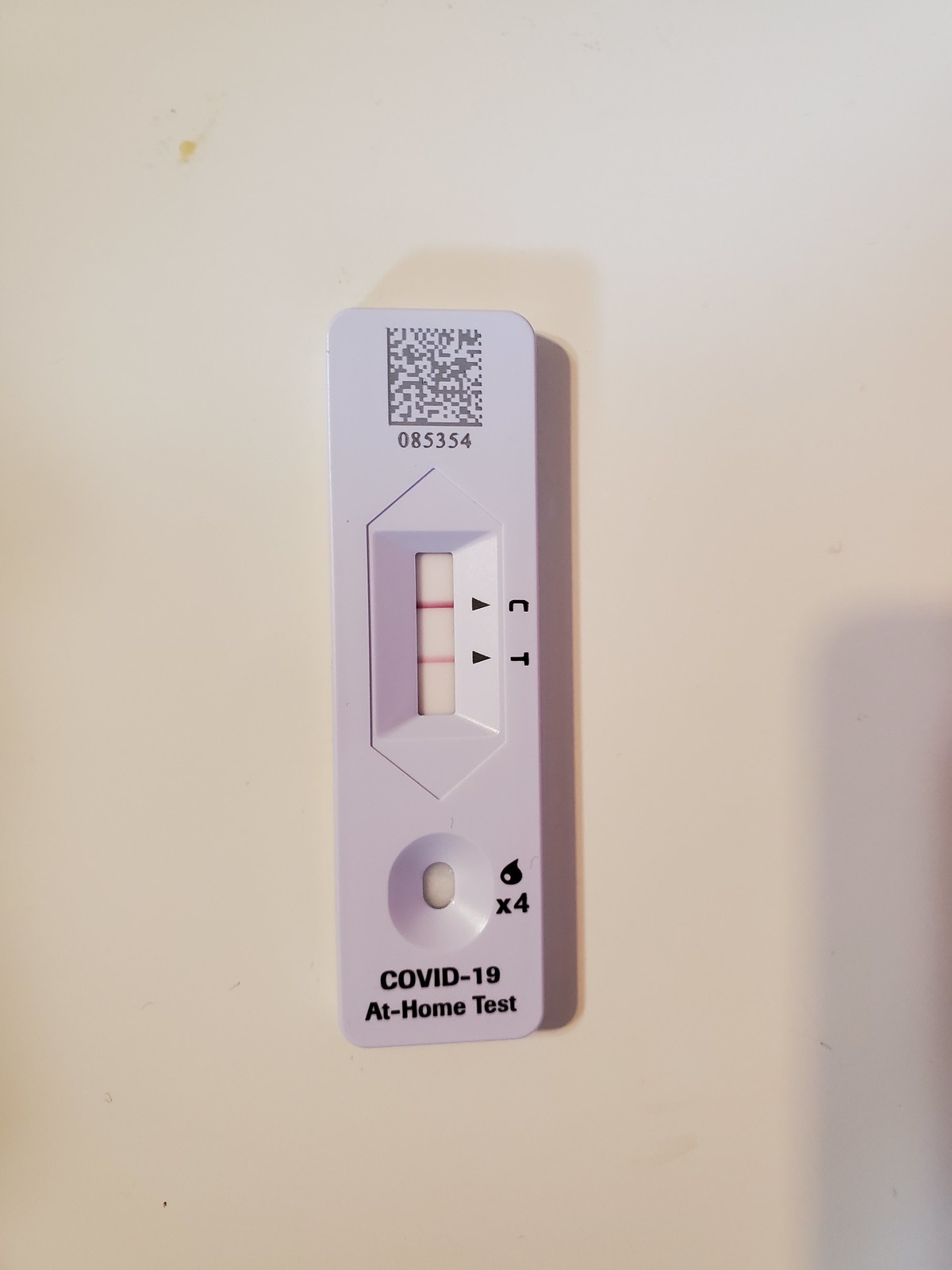A familiar sight during the COVID-19 pandemic, this image features an at-home COVID-19 testing kit. The rectangular white device prominently displays two slots: an oval application slot at the bottom and a rectangular result slot at the top. The test has been used, as indicated by the presence of fluid in the application slot where a sample swab was deposited. In the result slot, the control line is a vivid red, confirming the test's validity. Next to it, a second red line, albeit lighter in intensity, has appeared at the test marker (T), indicating a positive result. This nuanced shading reflects the possible intensity of infection. The detailed design and functionality of the kit make it an invaluable tool for quick and efficient home testing.